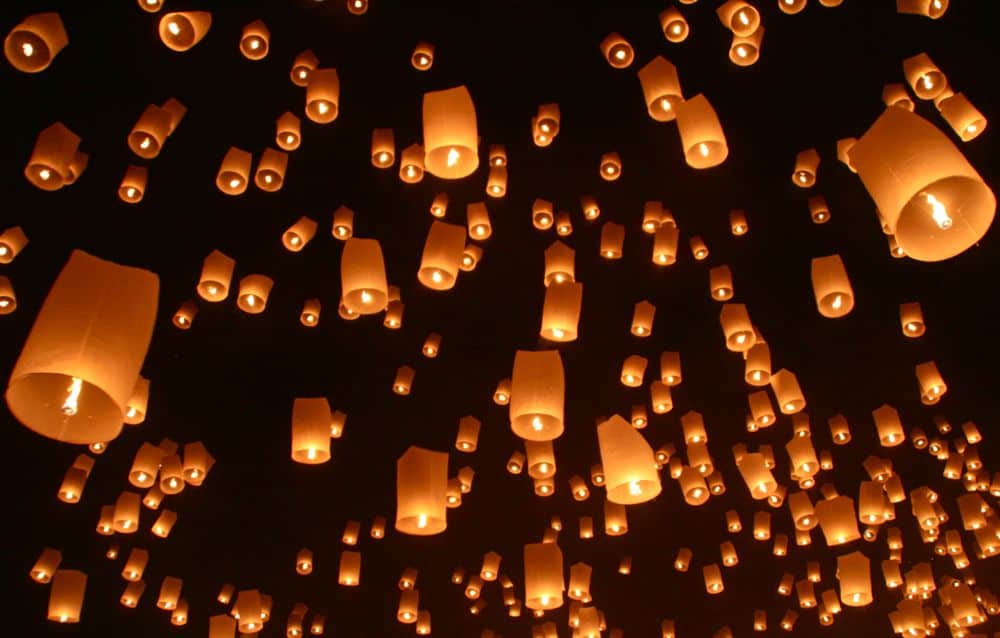The photograph captures a nighttime scene of numerous floating paper lanterns ascending into a dark sky. The image, taken from below, presents a wide rectangular view that emphasizes the vertical climb of the lanterns. Each lantern is cylindrical, taller than wide, and exhibits a light grayish-orange hue tinged with yellow near its base. The open bottoms of the lanterns reveal glowing flames that provide the lift needed for their flight. Closest to the camera, larger lanterns appear, including prominent ones in the left and top right corners. As the lanterns recede into the distance, particularly noticeable in the bottom right corner, they cluster more densely together and appear smaller. The overall effect is a mesmerizing cascade of lanterns, creating a spectacle of light against the dark expanse.